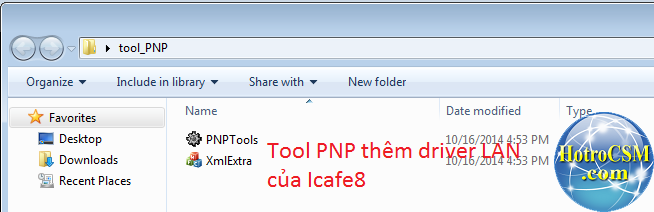This screenshot depicts a Windows directory window showing the contents of the folder "tool_PNP." The user interface has a gray background, typical of older Windows versions. At the top of the window, the title bar displays "tool_PNP." Below it, there are navigation options including left and right arrows, a drop-down arrow, and several tool options: "Organize," "Include in library," "Share with," and "New folder," each accompanied by a drop-down menu. 

On the left-hand side, the directory tree includes favorites with a star icon, "Desktop" with an associated desktop icon, "Downloads" with a blue arrow on a folder, and "Recent places" with a clock and paper icon. The main directory listing in the center of the window shows columns for "Name," "Date modified," and "Type." Notably, two items are listed: "PNP tools" and "XMLExtra," both modified on 10-16-2014 at 4:53 PM. 

Additionally, the image includes some red overlay text reading "tool_PNP," along with other text elements like "driver LAN" and "CUALCAFE8." There is also a blue orb featuring a website link near the right side of the window.